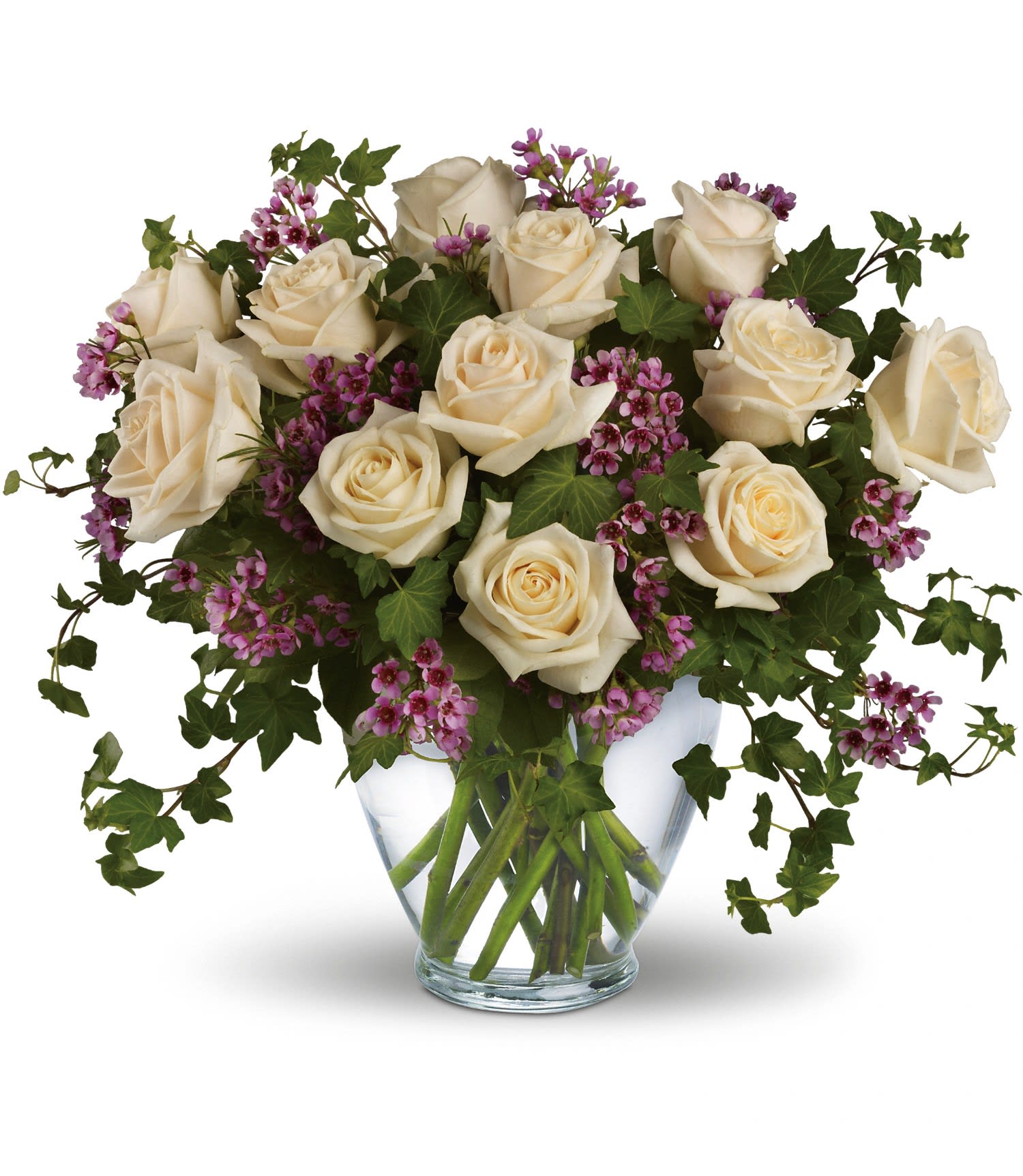This detailed photograph showcases a professionally arranged bouquet within a clear glass vase filled with water, set against a stark white background, suggesting a catalog or florist website listing. The centerpiece flutters with a dozen white roses, their pristine blooms surrounded by the natural greenery of leaves and stems. Interspersed among the roses are delicate sprigs of light purple flowers, each with hints of fuchsia at their centers, adding a subtle yet vibrant contrast. Additionally, vines weave gracefully throughout the arrangement, cascading over the vase's rim. The thin bottom of the vase widens at the top, allowing a pleasing spread of floral elegance. The overhead lighting casts a gentle shadow of the bouquet, enhancing the professional and serene presentation of the floral display.